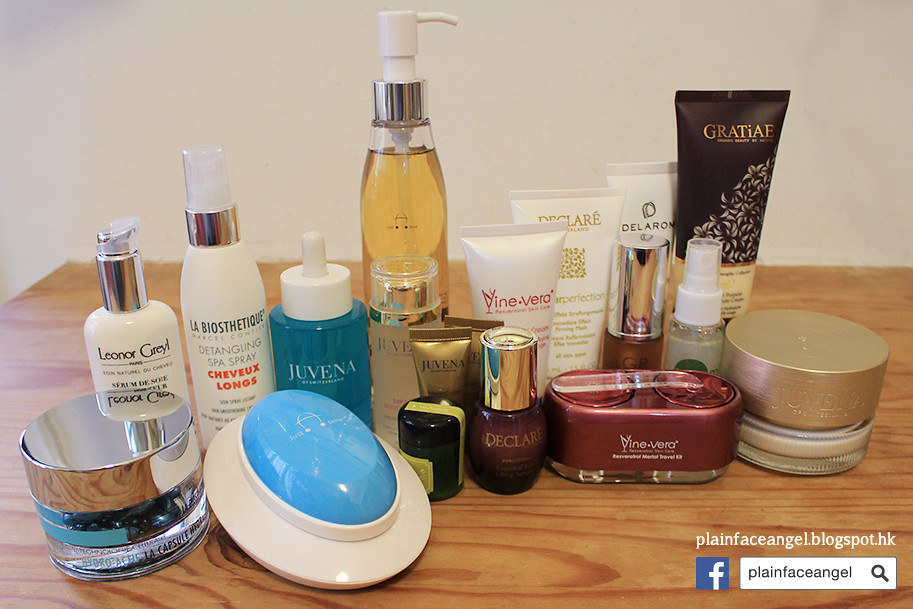This photograph, taken on a wooden table, features an array of personal hygiene and beauty products meticulously arranged. Starting from the left, you can see a glass circular container with a metallic lid, which holds face creams. Directly behind it is a cylindrical tube labeled "liner" or "grill," assumed to be a type of serum. Following that are four sequentially arranged serums for hair, which progress in color from white to a more yellowish-beige shade towards the center of the image.

From the center to the far right, there are four white tubes featuring various brand names. The far-right tube is black and branded as "Gratier." To the left of that is a white tube labeled "Deleram," followed by another white tube marked "Declaree." Next in line is a white tube from the brand "Vinovera."

In the foreground, additional makeup items from the brands mentioned earlier—Declaree and Vinovera—can be seen, completing this detailed display of beauty and personal care products.